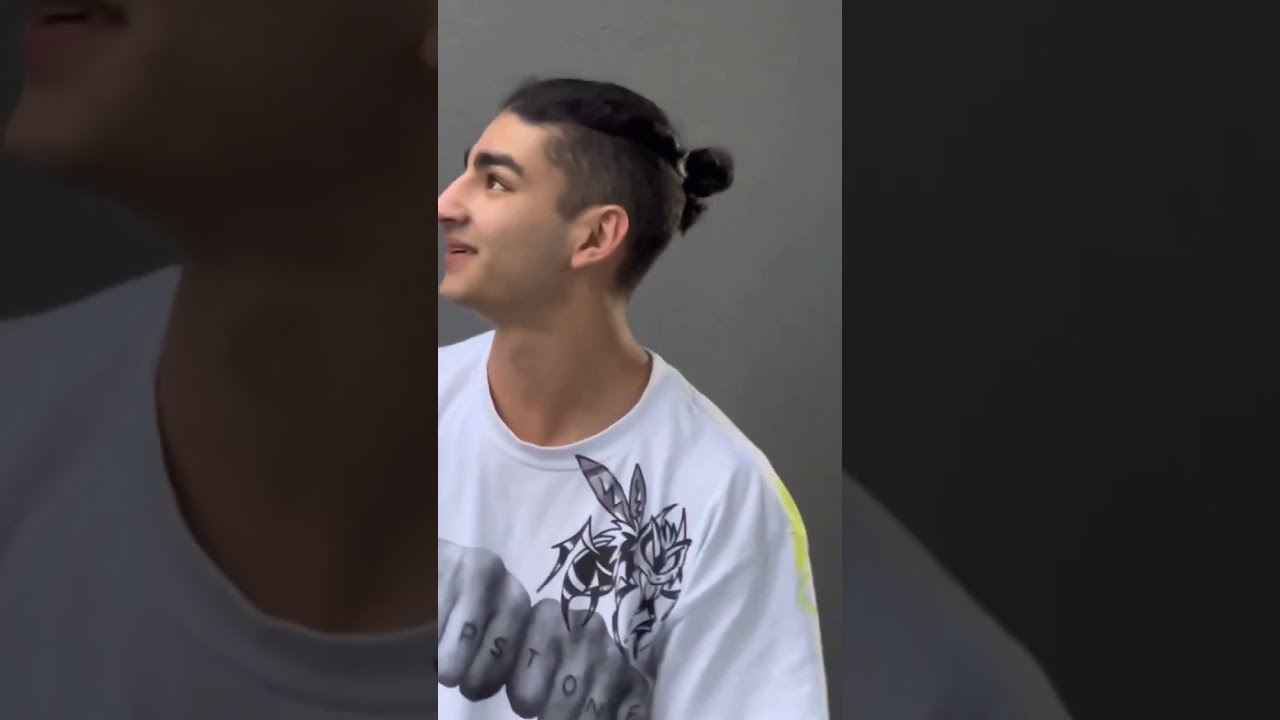This vertical photograph features a side profile of a young teenage boy, possibly around 16 or 17 years old, with dark, thick eyebrows and dark eyes. His hairstyle includes shaved sides and a small round bun at the back of his head. He is dressed in a white, somewhat baggy t-shirt that prominently displays an animated bee and a design of two fists with letters tattooed on the knuckles. The gray background contributes to the minimalistic setting. The boy’s nose tip is slightly cut off by the edge of the frame as he looks to his left, showcasing a hint of a smile. The left and right sides of the image are darkened and blackened out, emphasizing the central figure who appears to be preparing for a video presentation, possibly for social media like TikTok.